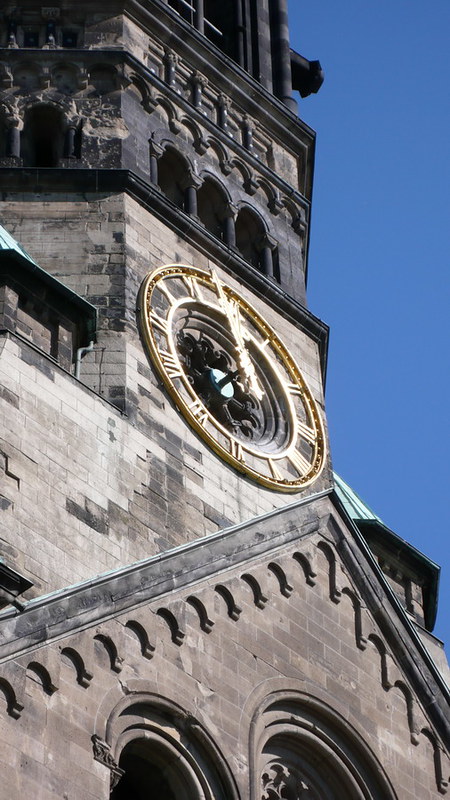The photograph captures an upward perspective of an old, Gothic-style church taken during the day against a clear blue sky. The church's weathered stone exterior exhibits a mix of black, gray, and lighter gray bricks, highlighting its significant age and intricate architecture. The building features two arched windows set within a triangular section at its base, giving it a grand and historic appearance. Toward the middle, there is an elaborate, gold-framed clock with prominent gold Roman numerals and gold minute and hour hands, which protrude on small black bars, reflecting sunlight to enhance visibility. Further up, a steeple with three additional arched windows can be seen, although the very top of the structure is cut off in the frame, suggesting a pointed peak extending out of view. Wooden or steel beams, discolored with age, add to the church's storied character.